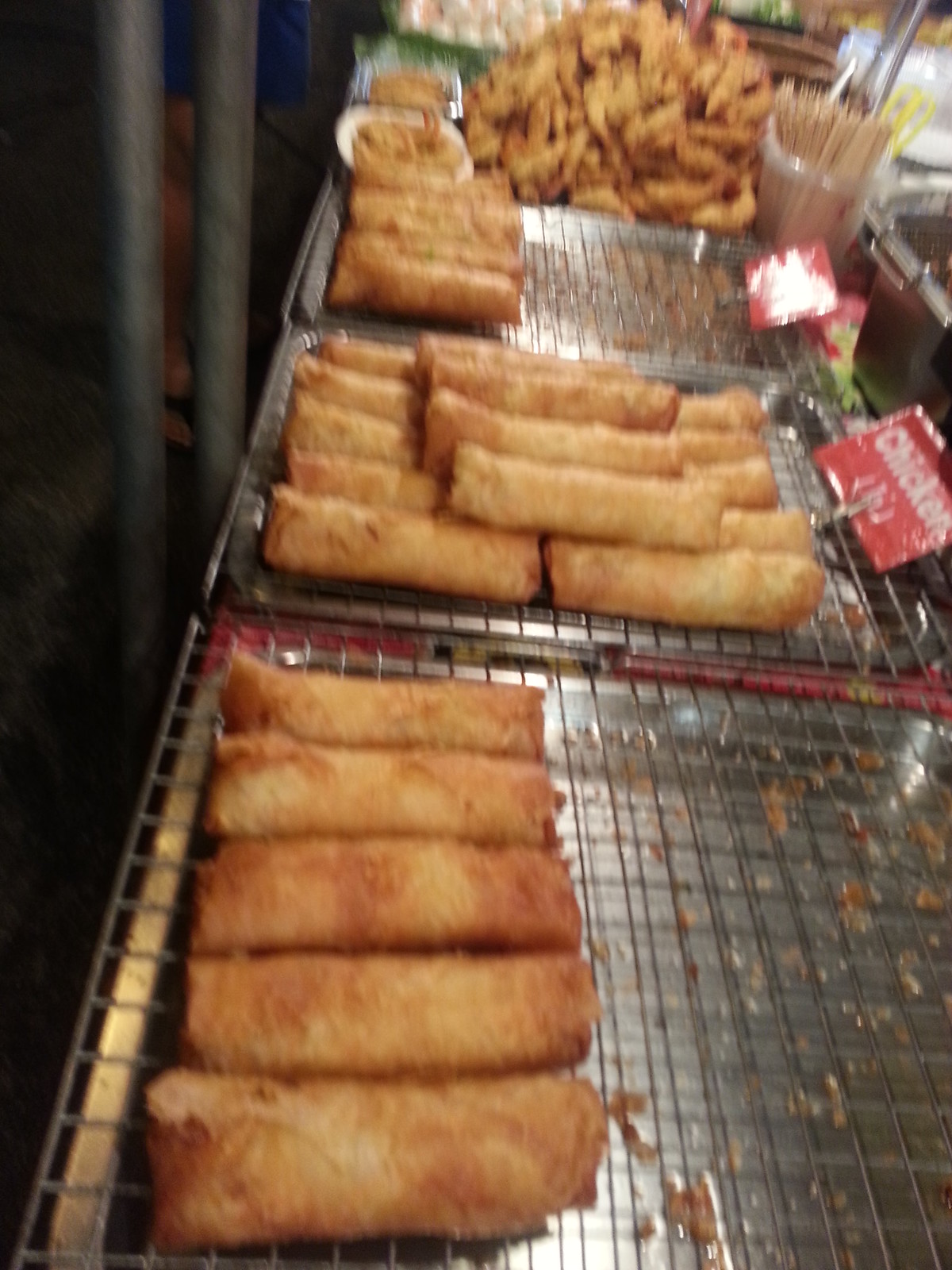The photograph shows an angled view of a section of a Chinese buffet, focusing on trays of egg rolls. The first three trays, each resting on gray grates over a large stainless steel pan, hold varying quantities of golden brown egg rolls. The tray nearest the camera has no visible sign and contains about five egg rolls. The middle tray, marked by a red sign indicating "chicken," holds a larger pile, around 15 egg rolls. The third tray also has a sign, although its writing is not discernible. In the background, a large pile of fried shrimp accompanies the egg rolls, and there's a plastic tub filled with chopsticks standing upright. In the top-left corner of the image, a portion of a black curtain is visible, contributing to the scene's casual, slightly out-of-focus ambiance.